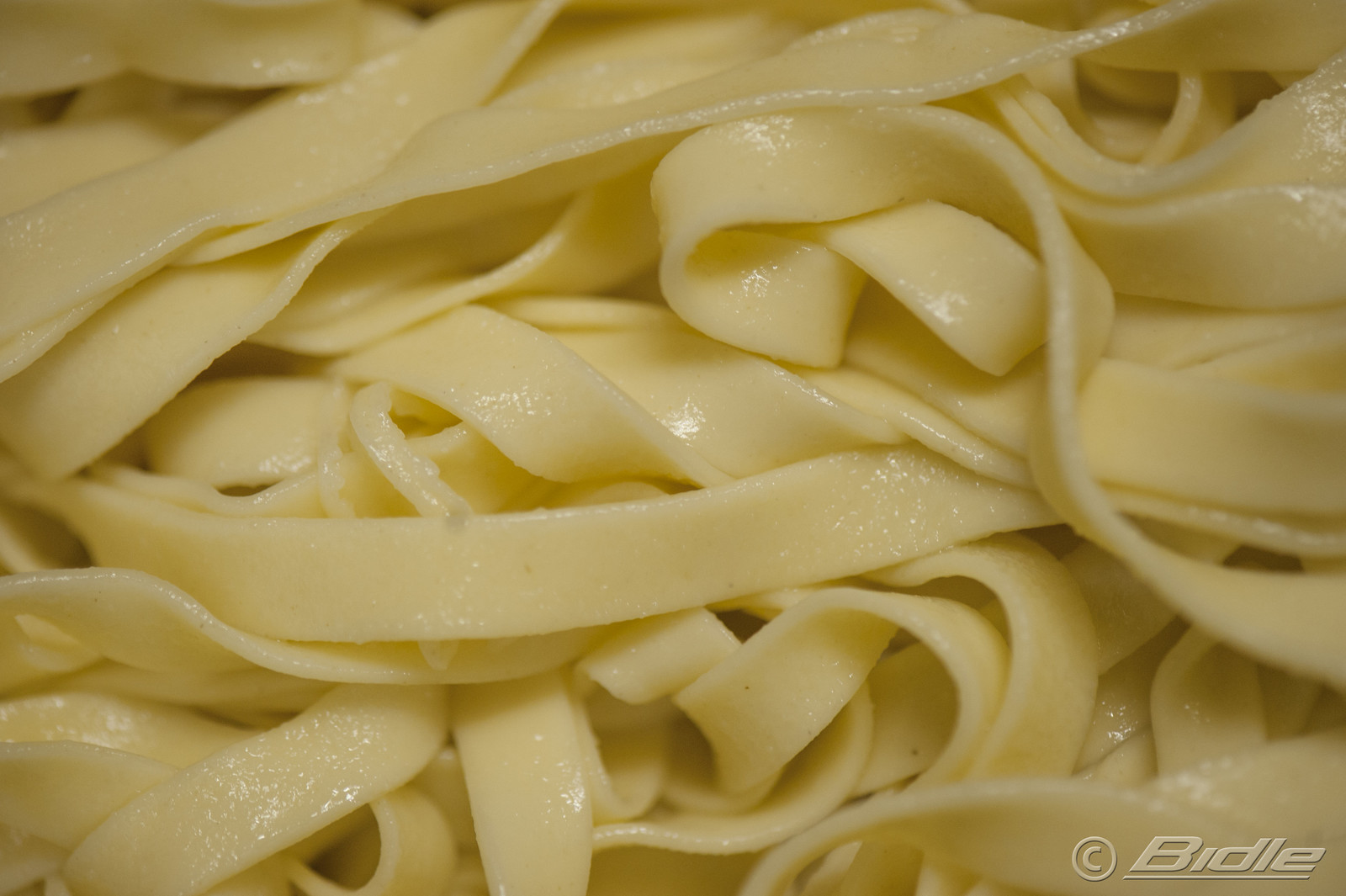This close-up image features a shiny, glossy bundle of fettuccine pasta noodles. The noodles appear to be freshly cooked, possibly straight out of boiling water or lightly coated with butter, giving them their sleek texture. The fettuccine, distinguished by its flat, ribbon-like shape, is randomly arranged with some strands straight, some curled, and others intertwined. The photo captures a high level of detail, showcasing the smooth texture of the pasta dough. At the bottom right of the image, the photo is marked with a copyright symbol and the underlined word "BIDLE".